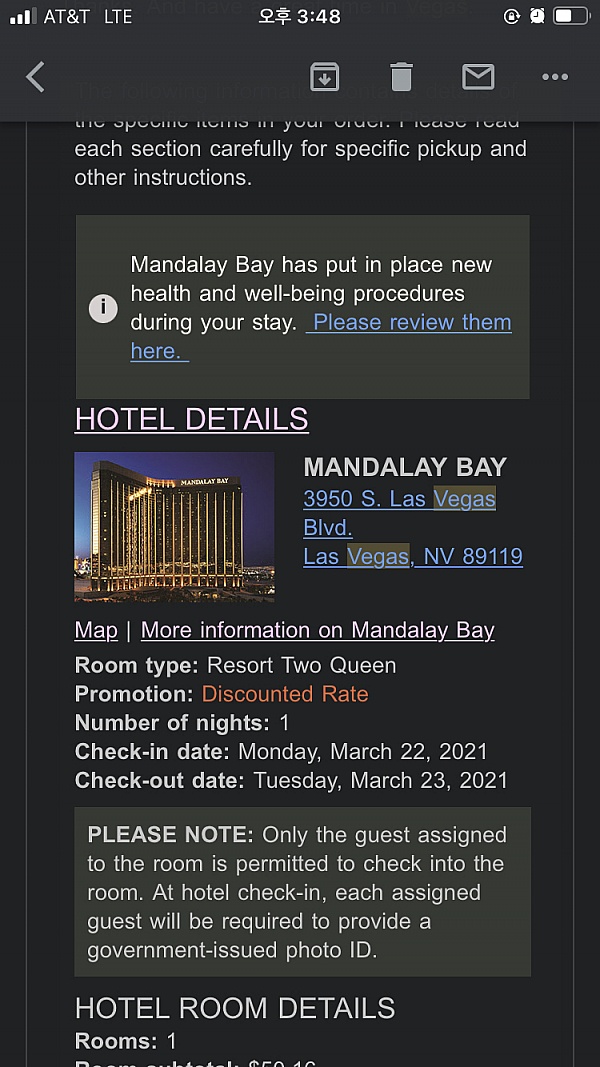The image captures a projection on a screen, set against a black background with predominantly white text. The screen appears partially unrolled, cutting off the top and bottom lines of text, making them unreadable. In the center of the screen, a picture of the Mandalay Bay Hotel is displayed. Directly below the image, the text reads: "Hotel details, Mandalay Bay, 3950 South Las Vegas Boulevard, Las Vegas." Additional links such as "map" and "more information on Mandalay Bay" are present. Above the hotel image, a message alerts guests that the Mandalay Bay has implemented new health and well-being procedures during their stay. In a prominent caption meant to catch attention, it advises: "Please note, only the guest assigned to the room is permitted to check into the room. At hotel check-in, each assigned guest will be required to provide a government-issued photo ID."